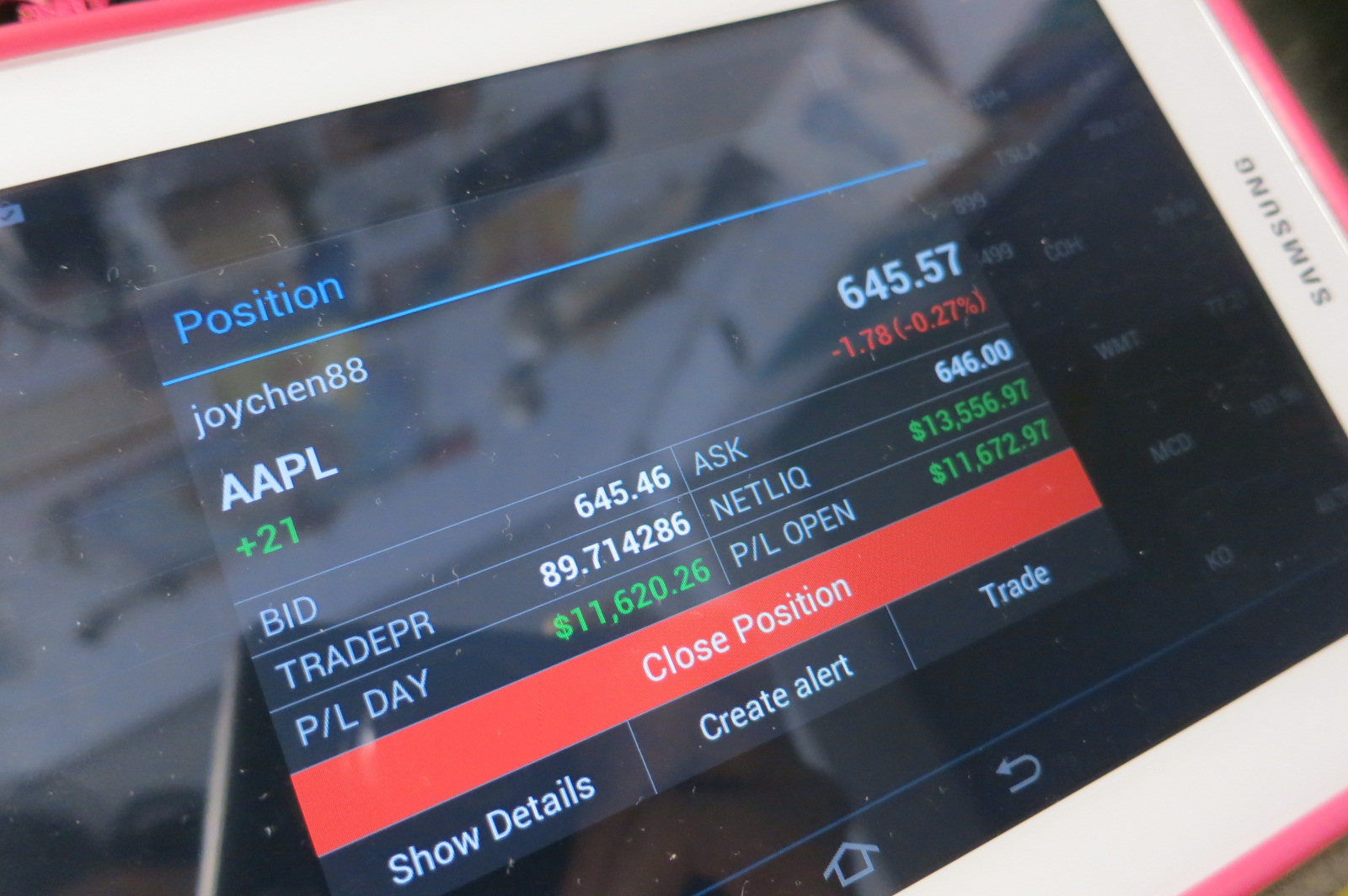This image captures a detailed view of a Samsung device screen displaying a stock market trading interface. The screen focuses on the stock for Apple Inc. (AAPL), showing a current price of 645.57, indicated as +21 in green. The display further details a decrease of 1.78 points or -0.27%. The bid price is 645.46, and the ask price is 646.00. There's a trade price of 89.714286, with a net liquidation value at $15,356.97 and a detailed position showing a daily profit and loss (P/L) of $11,620.26. The overall open profit and loss is $11,672.97. Prominently, there is a bright orange button labeled "Close Position," with additional options below it to "Show Details," "Create Alert," and "Trade." These elements collectively identify this screen as part of a trading platform interface used for monitoring and managing stock positions.